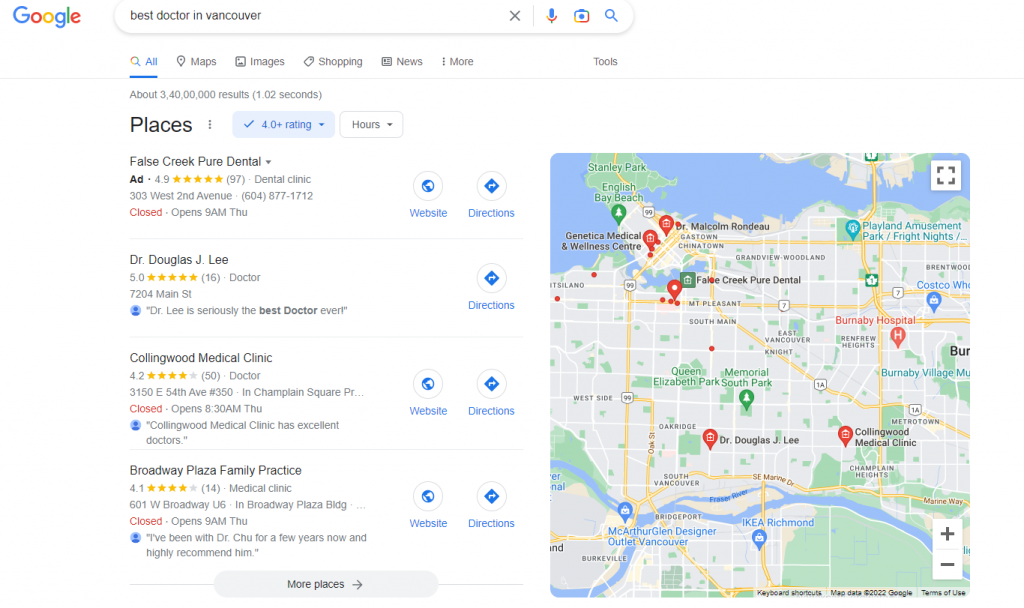The image displays a Google search results page with the query "best doctor in Vancouver" entered in the search bar. The search yields approximately 3.04 billion results in 1.02 seconds. Below the search bar, there are filter options highlighted in blue and red, allowing users to refine results by places with 4.0+ ratings and operational hours.

The first search result is an advertised entry for "False Creek Pure Dental," boasting a 4.9-star rating from 97 reviews. It's a dental clinic located at 303 West 2nd Avenue. The clinic is currently closed and will reopen at 9 a.m. on Thursday. The entry provides options for "Website" and "Directions," a common feature across all results.

The second result is for "Dr. Douglas J. Lee," who has a perfect 5-star rating from 16 reviews. He is located at 7204 Main Street and is praised as "seriously the best doctor ever."

The third result is "Collingwood Medical Clinic," rated 4.2 stars by 50 reviewers. It is a medical clinic located at 3150 54th Avenue H350 in Champlain Square. The clinic is currently closed. Reviews highlight that "Collingwood Medical Clinic has excellent doctors."

The fourth result is "Broadway Plaza Family Practice," with a 4.9-star rating. This medical clinic is situated at 601 West Broadway, Unit 6. The clinic is also currently closed, and a review mentions, "I've been with Dr. Chu for a few years now and highly recommend him."

At the bottom of the results, there is a "More places" option, and to the right side of the page, a map provides a visual aid for locating these medical services.